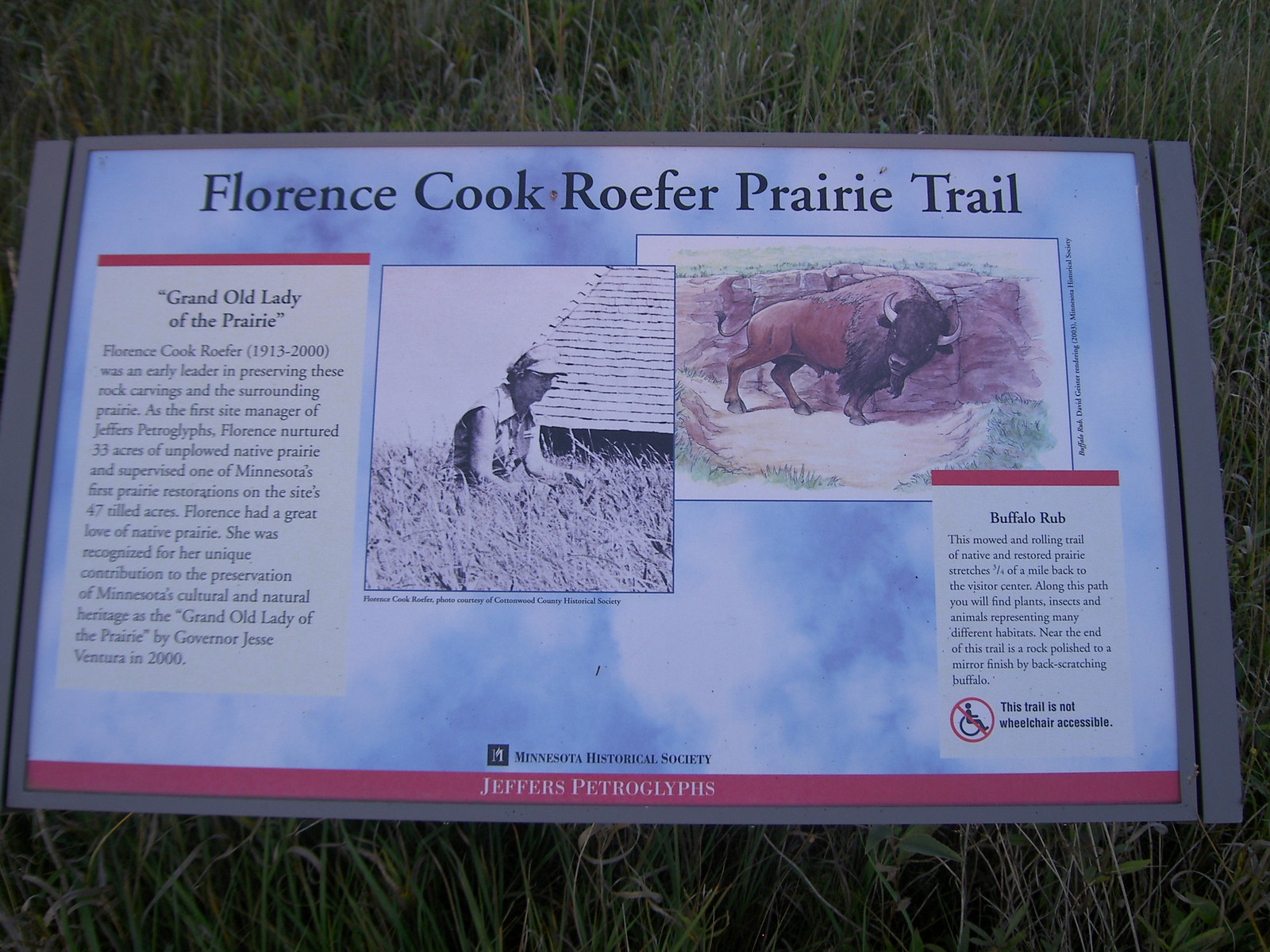This photograph captures an informative outdoor display situated against a lush, grassy backdrop. The display, laminated and framed with a gray wooden border, is set against a sky-blue background filled with white clouds. The header reads "Florence Cook Roefer Prairie Trail," followed by the subtitle "Grand Old Lady of the Prairie." This section provides detailed information on Florence Cook Roefer (1913-2000), heralding her as an early leader in the preservation of the rock carvings and native prairie at Jeffers Petroglyphs. She managed the site, overseeing its prairie restoration efforts and was recognized by Governor Jesse Ventura in 2000 for her unique contributions, earning her the affectionate title "Grand Old Lady of the Prairie."

Adjacent to this text is a prominent black-and-white photograph of Florence Cook Roefer herself, depicted in a grassy field with a cap on her head and a building structure visible in the background. Further to the right, the display features a colorful illustration of a buffalo standing before a rock outcrop, with additional buffalo in the background. Underneath this drawing, a section titled "Buffalo Rub" contains another paragraph of information, though it is harder to read due to the text's smaller font size. At the lower right, a symbol explicitly indicates that the trail is not wheelchair accessible.

At the very bottom of the display, a bold red stripe runs horizontally, marked with "Jeffers Petroglyphs," and above it is the logo of the Minnesota Historical Society, indicating the origins and custodianship of this historical marker.